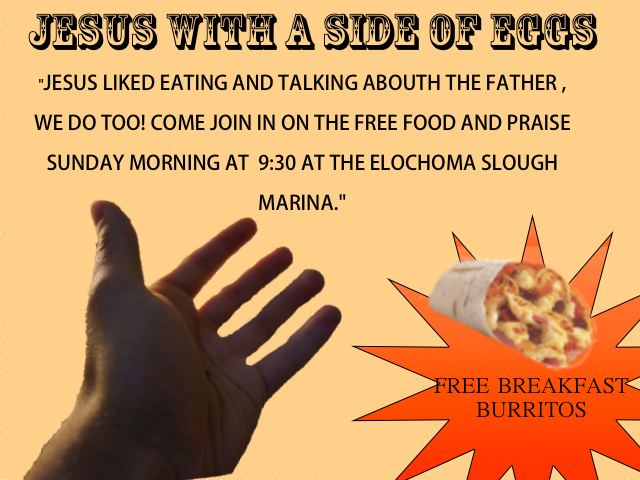The promotional graphic features a light orange background with an actual outstretched hand in the lower left corner reaching towards the center, where a pixelated image of a burrito is displayed inside a starburst-shaped graphic with an orange and red gradient. In the bottom right corner, the text "Free breakfast burritos" is prominently shown beneath the burrito. Across the top of the image, bold text reads, "Jesus with a side of eggs," followed by a quote: "Jesus liked eating and talking about the Father. We do too. Come join in on the free food and praise Sunday morning at 9:30 at the Elokoma Slough Marina."